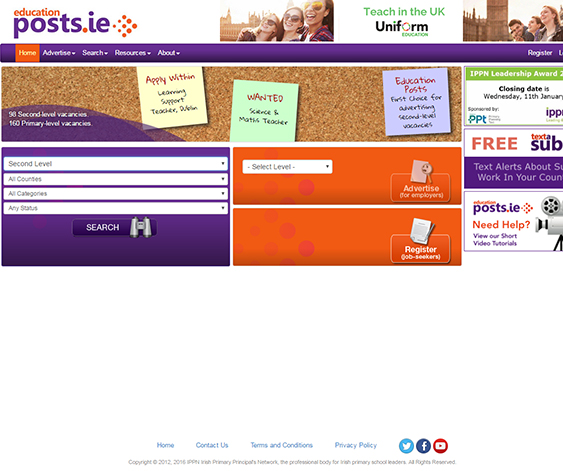This screenshot depicts the homepage of the website "educationposts.ie," a platform presumably related to education resources and job postings. The website's logo is located at the top left corner, featuring a small orange "education" text placed above a larger purple "posts.ie," with the dot in ".ie" also colored orange. Adjacent to the logo, an array of smaller dots transitions into larger ones, forming a diamond shape.

Directly below the logo is a purple navigation bar with labeled tabs: Home, Advertise, Search, Resources, and About. The 'Home' tab is currently highlighted in orange, indicating the active page. Above the navigation bar, there appears to be an advertisement or a promotional banner touting "Teach in the UK Uniform Education." This section includes images of what seem to be college students sitting outdoors against the backdrop of an iconic London building.

Beneath the navigation bar, there's an image of a table scattered with sticky notes of various colors: yellow, green, and purple, each containing distinct messages. This colorful display adds a vibrant and organized feel to the webpage layout. The overall design and structure of the website blend informational and visual elements seamlessly.